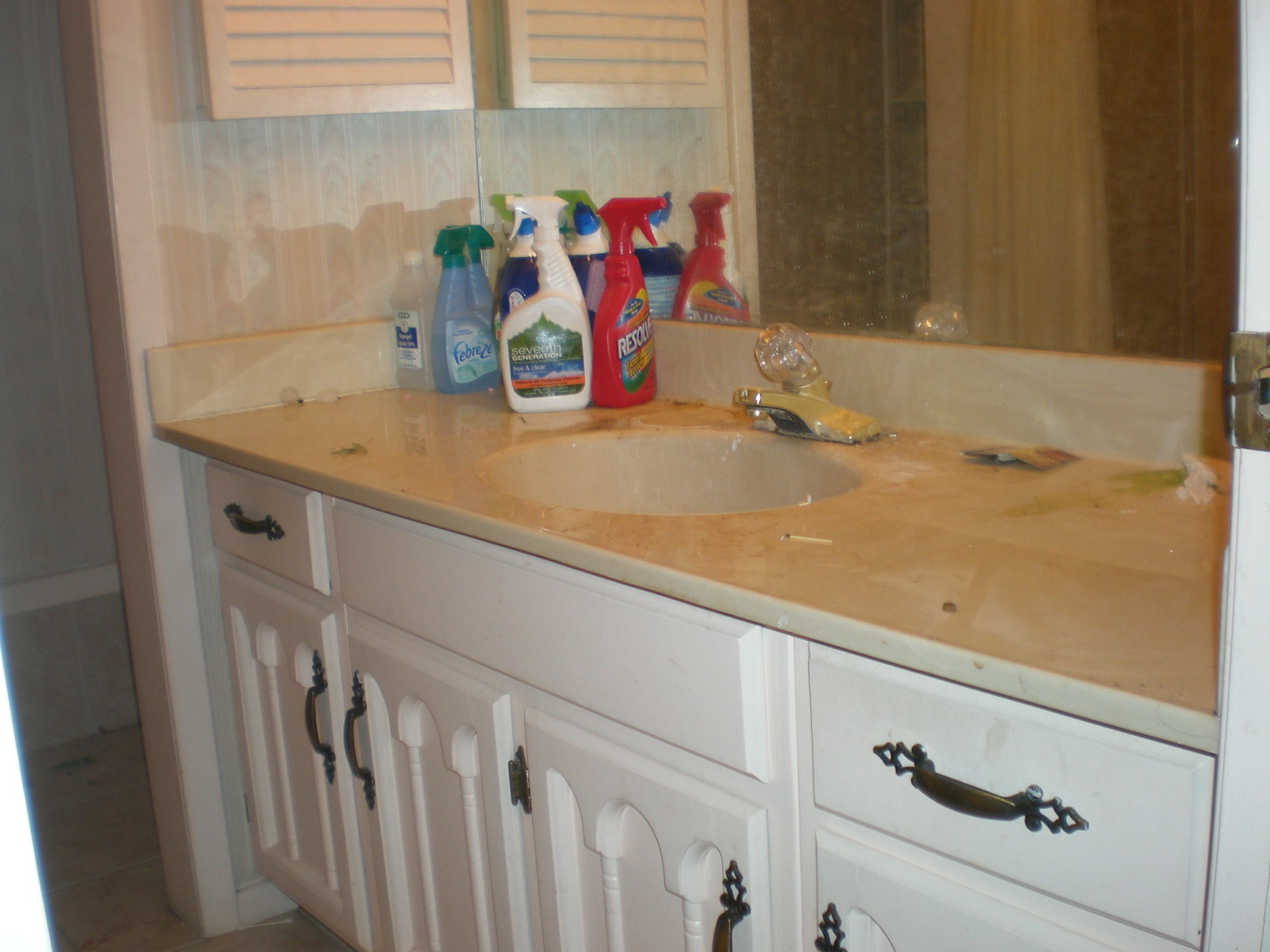The image depicts a rather dated bathroom scene. On the right side, part of a large mirror is visible, reflecting portions of brown walls in the background. Adjacent to the mirror, there is a peach-colored shutter, only partially visible with its bottom reflected in the mirror. The bathroom features dated wallpaper adorned with muted, vertical peach stripes. To the left, there's a doorway framed with white molding.

The bathroom sink area is showcased prominently, featuring a long and narrow countertop also in a peach hue. The sink is outfitted with a clear, push-up handle for water control and is accompanied by a silver faucet. Reflected in the mirror are various cleaning supplies: a red bottle of Resolve facing right, a white Seventh Generation bottle centered and facing left, a blue bottle of Febreze, and what appears to be a bottle of rubbing alcohol.

The counter extends to a corner next to the mirror, and below it, white cabinets with bronze handles and a couple of drawers at the top provide storage, contributing to the somewhat antiquated aesthetic of the space.